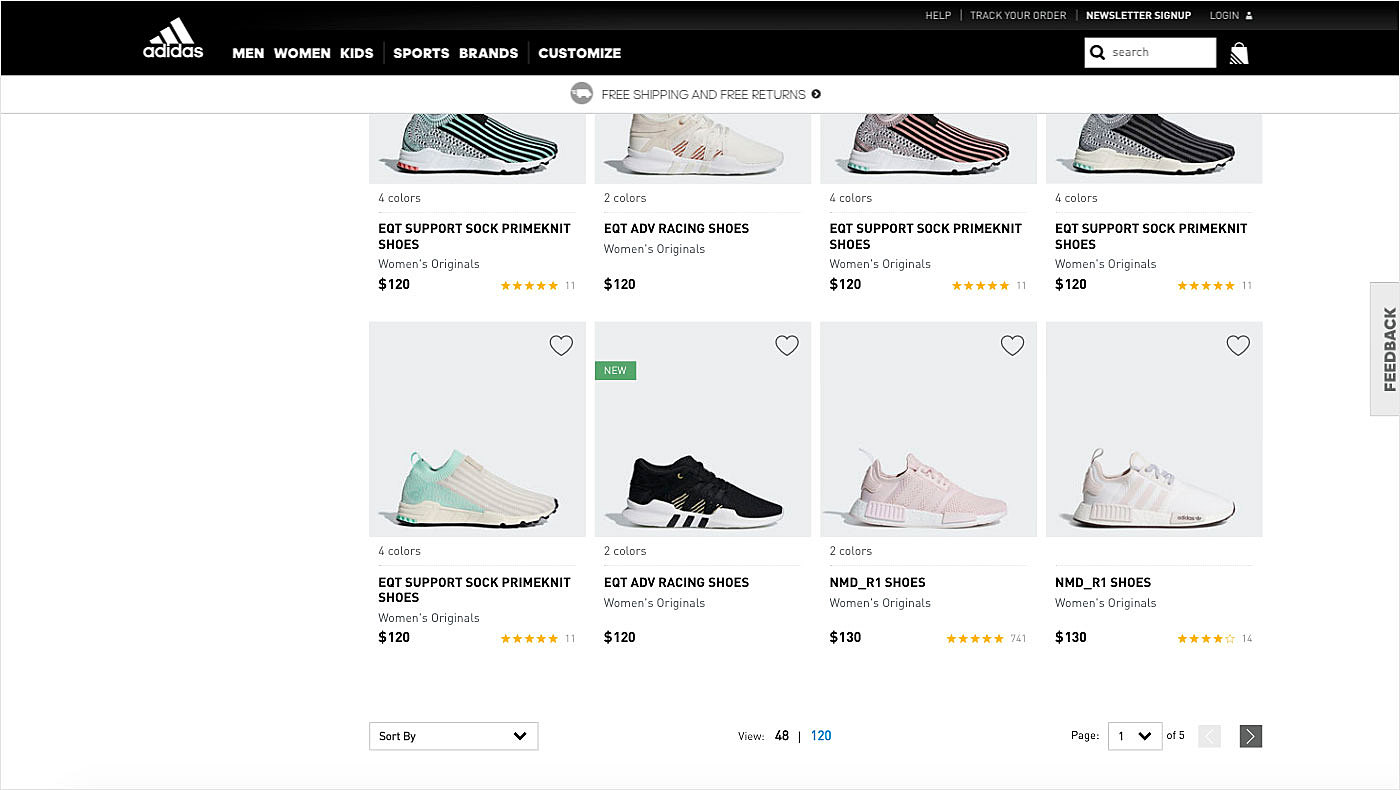The image displays a results page on the Adidas website. In the upper left-hand corner, the iconic Adidas name and logo are prominently featured. A black navigation bar stretches across the top of the page, with bold white text offering various categories: Men, Women, Kids, Sports, Brands, and Customize. Towards the right, the black bar includes a search bar and a shopping bag icon. At the very top, a smaller menu presents options for Help, Track Your Order, Newsletter Signup, and Login.

Beneath the navigation bar, the page highlights a promotional banner for Free Shipping and Free Returns. Below this banner, there are images of eight different types of shoes. Each shoe image is accompanied by a product description, price, and user ratings. An empty heart icon appears in the upper right corner of each shoe image, allowing users to favorite the item.

At the bottom of the page, a drop-down menu labeled "Sort By" enables users to arrange the listed shoes according to various criteria. Another option allows viewers to choose how many items are displayed per page, either 48 or 120. Finally, a drop-down menu on the far right lets users navigate through different page numbers.